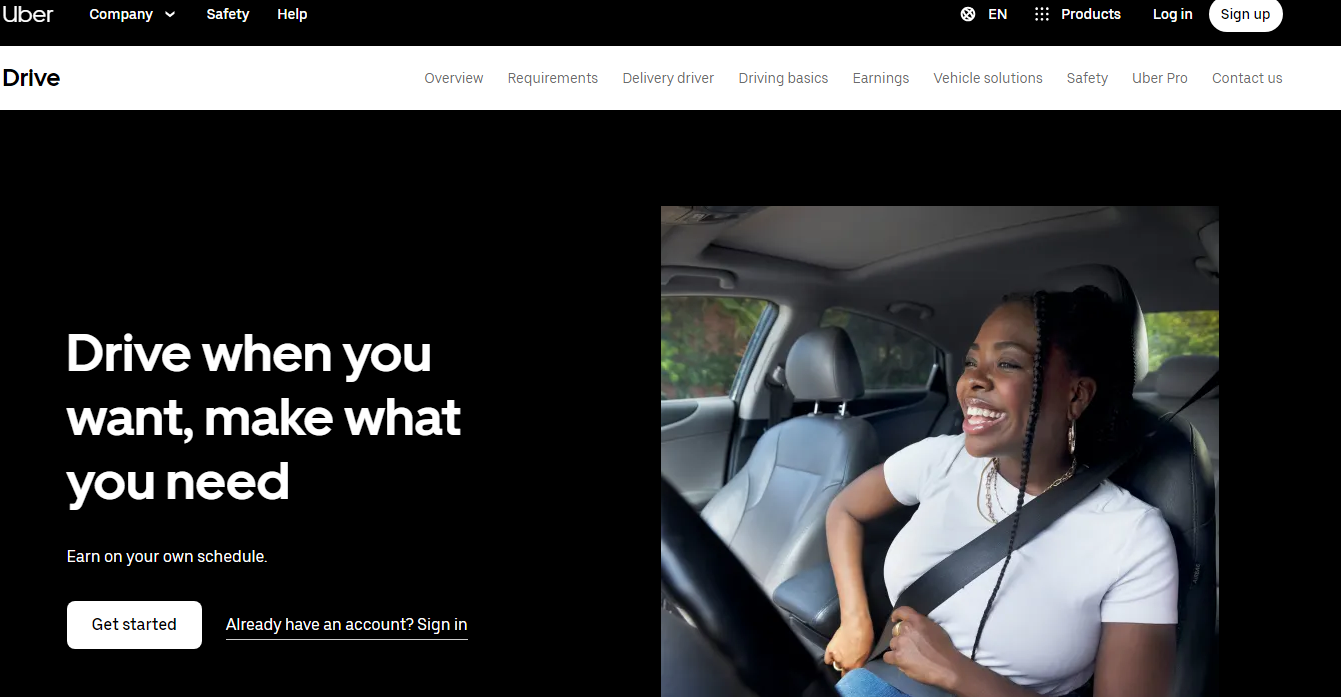Screenshot of Uber Homepage:

At the top of the screenshot is a black navigation bar with white text, featuring the Uber logo on the far left followed by links labeled "Company" with a downward arrow, "Safety," and "Help." The text "EN" indicates the website's language setting. To the far right, links to "Products," "Log in," and "Sign up" are displayed.

Beneath the black bar, a white secondary navigation bar contains additional options for drivers, including "Drive," "Overview," "Requirements," "Delivery Driver," "Driving Basics," "Earnings," "Vehicle Solutions," "Safety," "Uber Pro," and "Contact Us."

The main section of the screenshot is dominated by a promotional banner with a black background. On the right side is an image of a young Black woman with a wide, friendly smile, sitting in her car. She is wearing a white t-shirt and blue jeans and is in the process of fastening her seatbelt.

To the left of the image, a bold white text reads: "Drive when you want, make what you need, earn on your own schedule." Below this tagline is a white "Get Started" button with black text. Further down, smaller white text on a black background invites existing users to "Already have an account? Sign in."